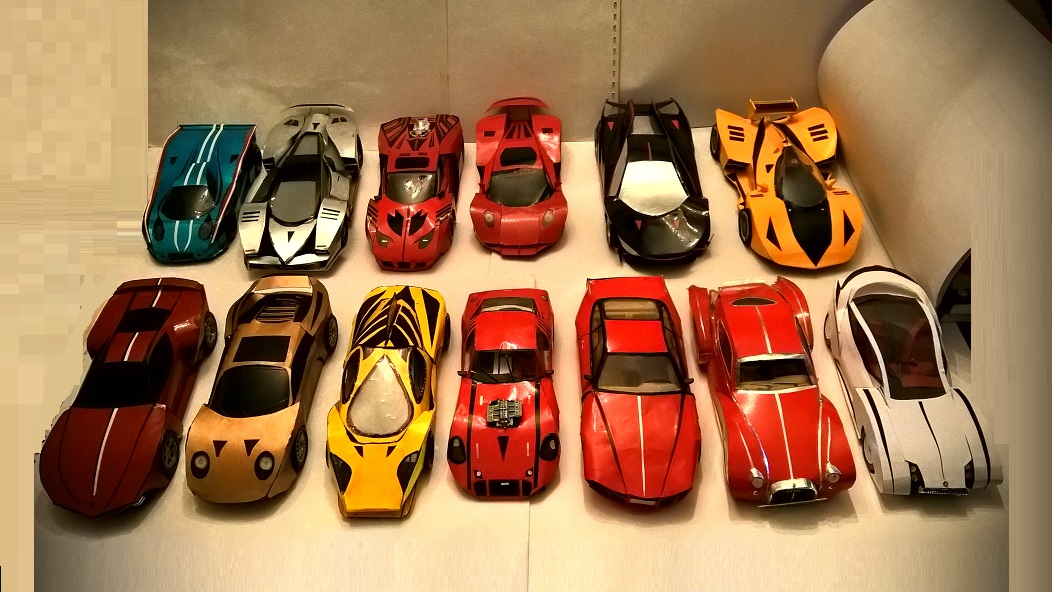This low-light photograph showcases a collection of 13 toy cars arranged on what appears to be an off-white, possibly leather chair. The cars are organized in two rows. In the back row, six cars face forward, starting with a greenish-blue car on the top left, followed by a silver sports car resembling a Lamborghini. Next is a red car with black spots, another red sports car, a black sports car, and a yellow sports car with a black middle stripe. The front row features a maroon-colored car, then a gold car, followed by a yellow car. Further to the right are three consecutive red cars, and finally, a bright white car. The cars vary in style from futuristic and modernized classic race cars to ones reminiscent of older models, including potentially 1920s design, with vibrant colors and accents that include black or silver trims and stripes.